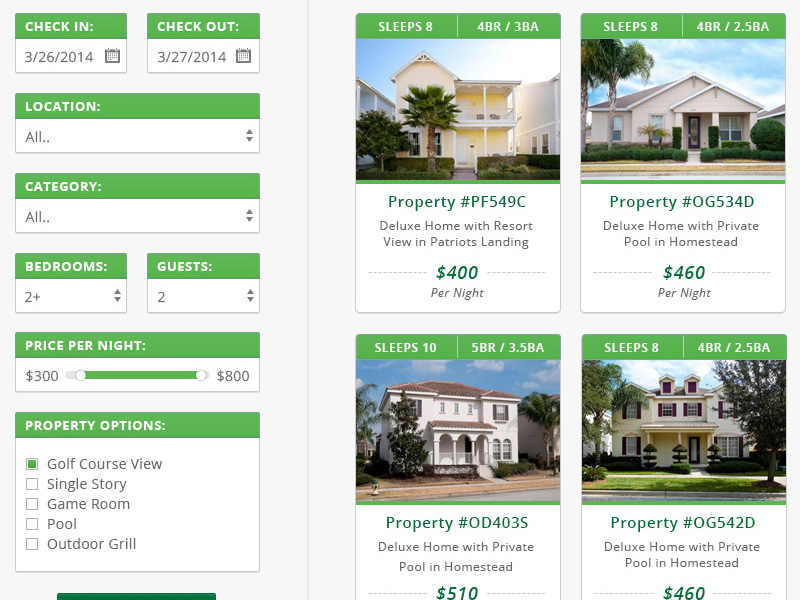This image is a web interface designed for renting a house by the night. On the left-hand side, there are check-in and check-out options, highlighted in green text with a white background. The check-in date is set to March 26, 2014, and the check-out date is March 27, 2014; both dates are accompanied by small calendar icons. Below these options is a drop-down menu for selecting a location, with "Location" written in green text and "All" displayed in black text within a white background. 

Following this is another drop-down menu for selecting a category, which is also set to "All." Further down, there are options to specify the number of bedrooms (2+) and guests (2). The price per night section features an adjustable bar, which is currently set with a minimum of $300 and a maximum of $800 per night.

Under the "Property Options" heading, there are five checkboxes labeled: Golf Course View, Single Story, Game Room, Pool, and Outdoor Grill. The Golf Course View option is selected.

On the right-hand side of the interface, there are four images of properties available for rent:
1. The first property sleeps eight people and has four bedrooms and three bathrooms. It is priced at $400 per night.
2. The second property also accommodates eight guests, with four bedrooms and two and a half bathrooms, priced at $460 per night.
3. The third option sleeps ten guests and includes five bedrooms and three and a half bathrooms, with a nightly rate of $510.
4. The final property displayed sleeps eight guests, featuring four bedrooms and two and a half bathrooms, priced at $460 per night.